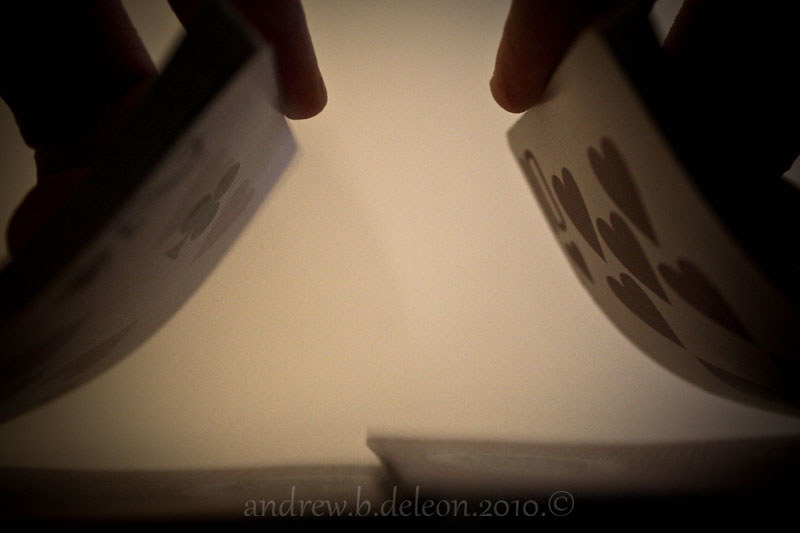In this detailed close-up image, we observe the intricate action of someone shuffling a deck of cards. The camera appears to be positioned very close to the table, capturing the motion from a low-angle perspective. Prominently, the copyright text "andrew.b.dillon.2010" is centered in the middle of the image. At the top portion, two hands are visible, each grasping a separate pile of cards, preparing to interleave them. Towards the bottom, we see the backs of several cards as they begin to cascade onto the table. On the right-hand side, a red Ten of Hearts card is distinctively visible. Contrastingly, on the left, the blur of motion obscures the exact identity of the cards, though there’s a hint it could be a black Two of Clubs. The entire scene unfolds against a backdrop of a tan or off-white-colored wall.